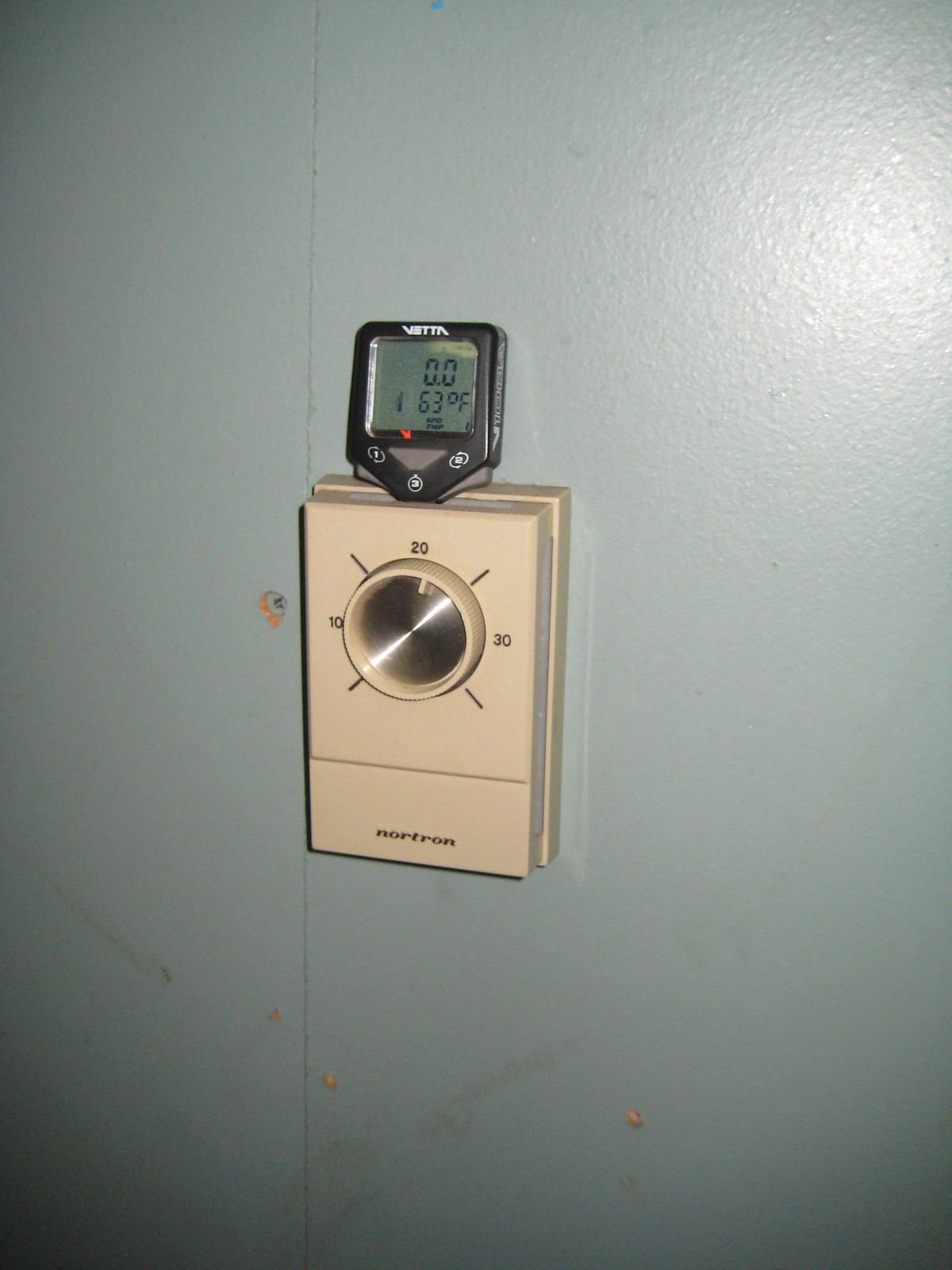The image depicts a thermostat mounted on a somewhat dirty, gray-colored wall, suggesting an indoor setting of uncertain location. The beige-colored thermostat occupies the middle section of the photograph. Prominently, a circular dial with a silver center is situated in the thermostat's middle. The dial is marked with temperature indicators: "20" at the top, "10" to the left, and "30" to the right. Additionally, small lines are positioned at each corner—top left, top right, bottom left, and bottom right—on the dial.

The brand name "Nortron" is inscribed at the bottom of the thermostat, indicative of its manufacturer. Atop the thermostat sits a black square device that narrows to a point at the bottom. This modern-looking device features a small digital screen that reads "0.063 degrees F," presumably providing a precise temperature reading linked to the thermostat. The contrast between the aged appearance of the thermostat and the newer digital device suggests the latter may have been added at a later time to enhance functionality. The overall impression is one of a well-utilized, perhaps older, temperature control system attempting to keep current with additional contemporary measurements.